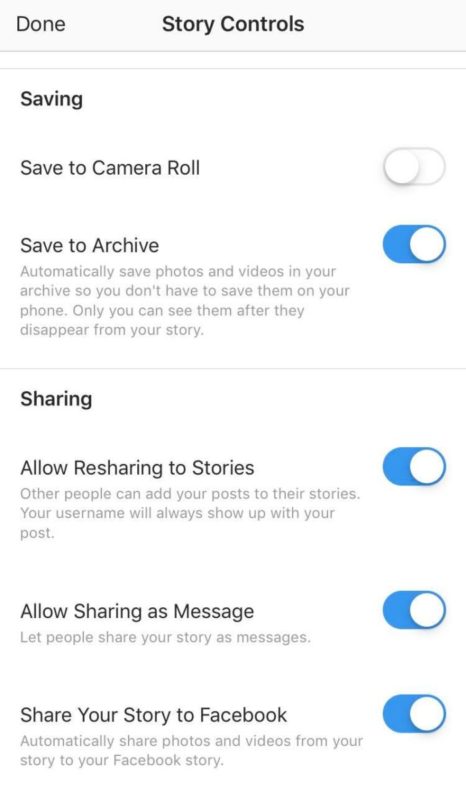This image depicts a phone interface with various storage and sharing options, likely from a photo application. At the top, the screen displays the button "Done" and the heading "Storage Controls." Below, a list of options includes "Save to Camera Roll," "Save to Archive," among others. Notably, "Save to Archive" is activated, indicated by a highlighted selection.

The description clarifies that saving to the archive automatically stores photos and videos in a separate archive, keeping them off the main phone storage but accessible to the user even after they disappear from a story. This feature is useful for preserving content privately.

A dividing line in the middle separates the storage options from the sharing options. The sharing section includes toggles for "Allow Resharing to Story," "Allow Sharing as Message," and "Share Your Story to Facebook," all of which are currently enabled. The only disabled option is "Save to Camera Roll."

The UI and UX design of the interface suggest it is from an iPhone, given its clean and readable layout.